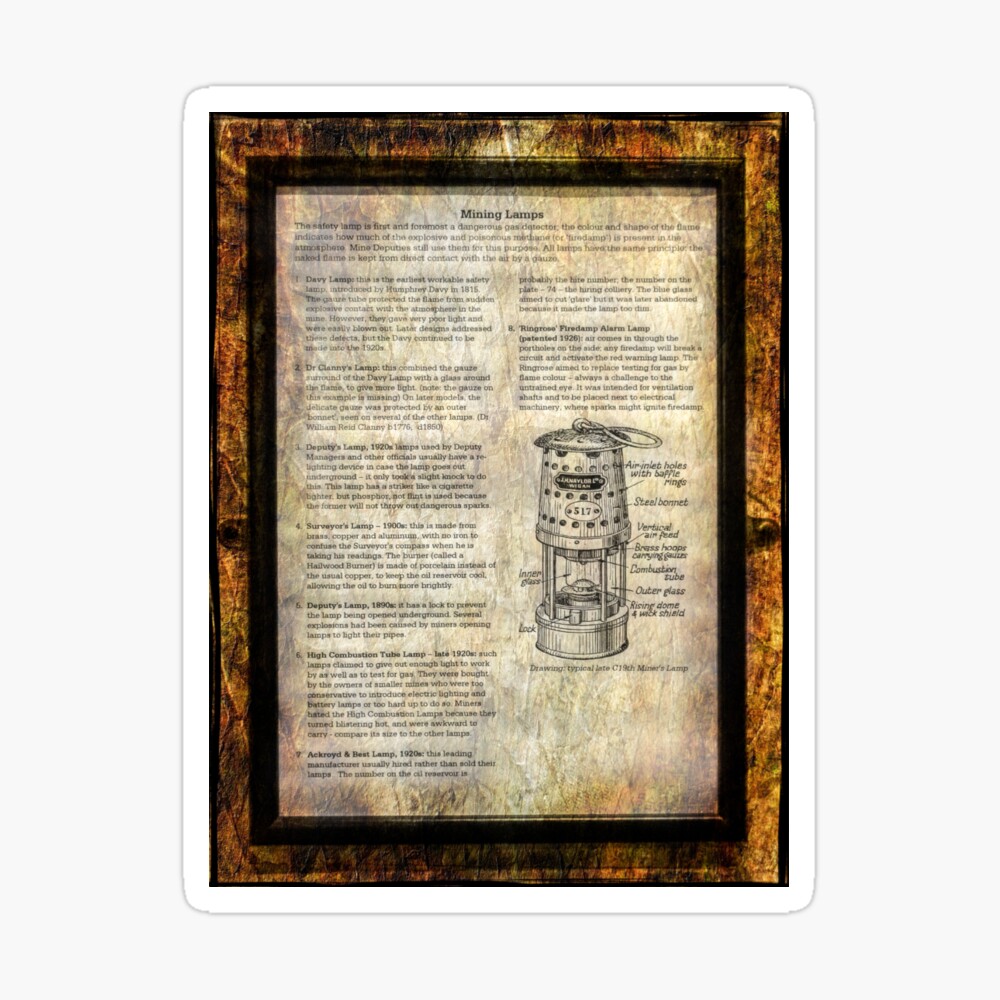The image is a detailed, framed photograph of an antique page from a book, specifically focusing on different types of mining lamps. The central page, which has the title "Mining Lamps" at the top, appears aged, with shades of yellow, beige, tan, and brown around its edges, giving it a vintage look. This page is bordered by a black frame, outside of which lies another border with a wood-like texture in warm tones of brown, orange, red, and light yellow. Surrounding this is a thin black border, all encased within an outermost white frame.

The page itself includes an intricate diagram illustrating a typical late 19th-century miner's lamp, complete with labeled parts like the bonnet, air inlet, inner glass, and lock. The lamp is described as having a ring on top for carrying, a perforated barrel that likely allows light to escape, and a section below for the flame, with a fuel compartment beneath, resembling a metal tin canister.

Though the surrounding text on the page is difficult to read from afar, it discusses the crucial role of mining lamps as safety devices, used primarily for detecting dangerous gases. The text seems to reference the evolution and various types of mining lamps, including mentions of figures like Debbie and Dr. Clanny, and details how these lamps functioned to counteract explosive and poisonous gases found in mines. The page ostensibly provides a guide to understanding the different lamp designs and their corresponding safety features, listing and illustrating eight specific lamp types in total.